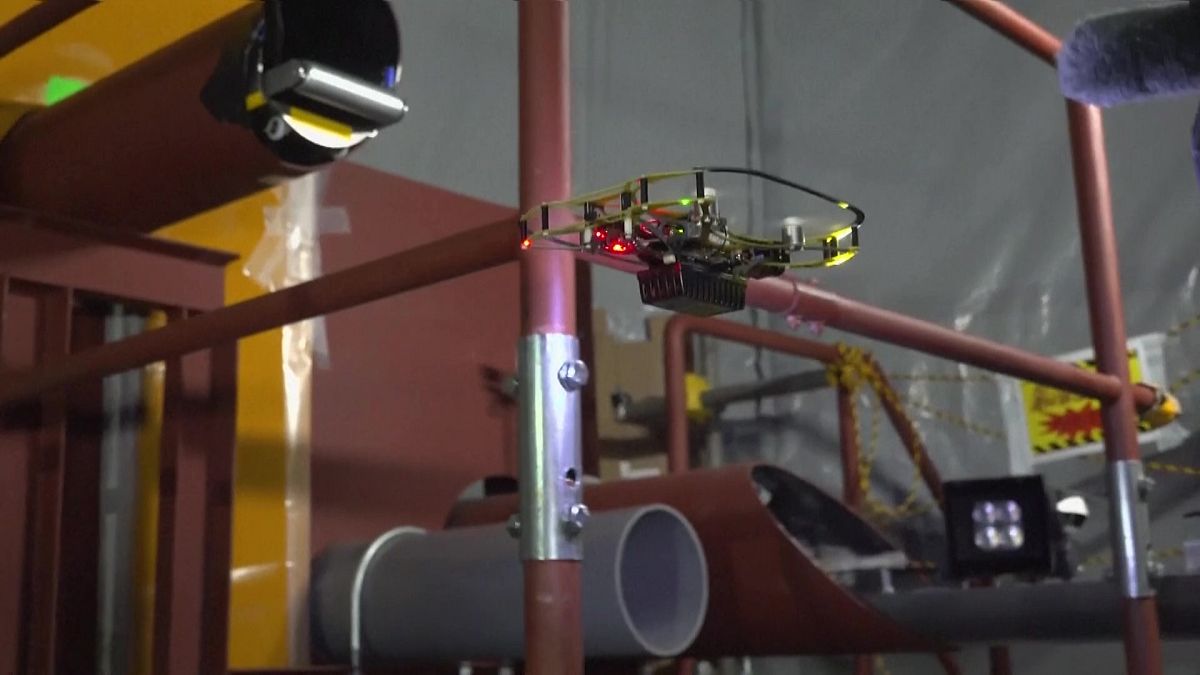The image depicts the interior of a factory or warehouse featuring an intricate assembly of machinery and metal piping. Central to the scene is an arrangement of dark red pipes, connected by steel rivets, with some sections extending vertically and horizontally. At the bottom of the image, there are gray tubes. The focal point of the machinery includes a gold-colored component with wire frames that don't seem to be connected to much and a rectangular part at its base. Toward the upper left, a pipe fitted with a valve leads to a yellow and silver contraption. 

In the background, there are bare gray walls with a slightly blurry caution sign positioned towards the right. The sign, featuring a yellow background with a red spiky symbol, is bordered by black and yellow diagonal stripes. Additionally, there's an indistinct purple and fuzzy object in the upper right corner that doesn’t appear to be part of the primary machinery setup. A closer look reveals scotch tape on the wall toward the left side of the image, adding to the scene’s industrial and somewhat disorganized atmosphere.